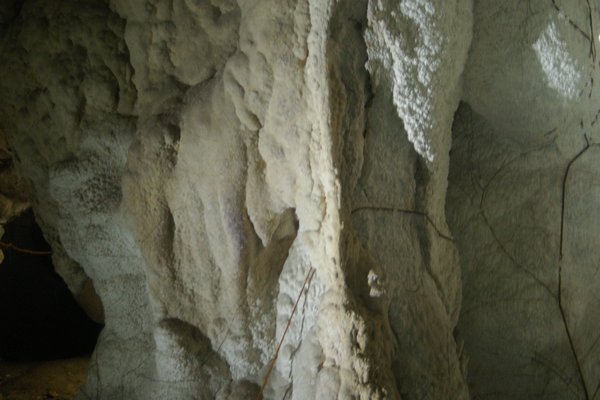The image depicts a close-up view of what appears to be the textured wall of a cave, predominantly featuring a light gray to white limestone surface with slight tan or beige hues in certain areas. The stone appears to have a varied texture that might be mistaken for coral due to its intricate details. Visible cracks accentuate its ruggedness, and the surface seems to grow darker towards the left and right edges, with a brighter section in the middle, possibly illuminated by an unseen light source. Towards the bottom left, there is an archway or opening suggesting a potential pathway deeper into the cave. On the right side of the image, there are branch-like formations, resembling skinny tree vines or possibly worn-out cables draped across the wall, adding to the natural yet mysterious feel of the scene. The overall color palette is muted, emphasizing the natural composition of the cave's interior.